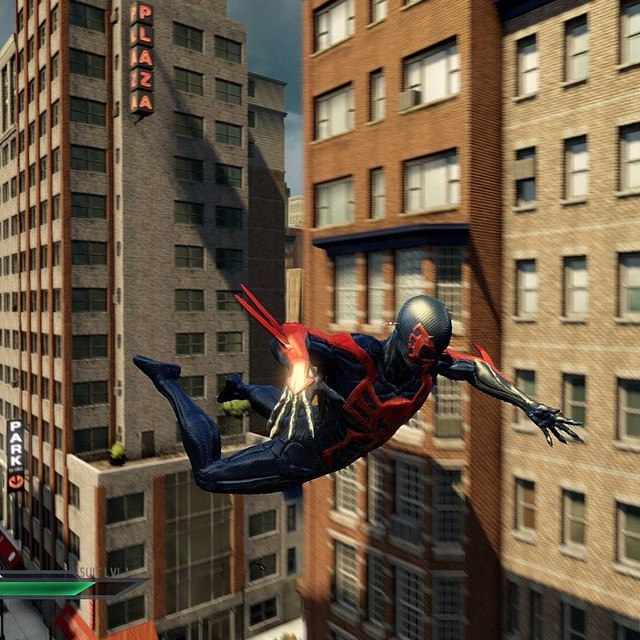The image depicts a highly detailed 3D render of Spider-Man 2099 soaring through a cityscape, likely in a scene from a video game. The character is shown in a dynamic leap from left to right with an athletic and muscular build. He is clad in a sleek black suit with red accents, including a red spider logo on his chest, arms, and face mask, which has a distinctive carbon fiber texture. The backdrop features towering brownstone buildings with numerous windows, highlighting an urban environment. At the top of one building, a neon sign reads "PLAZA" in illuminated letters, while another sign at street level indicates a parking area. The sky above is overcast with dark grey clouds, casting a moody atmosphere over the scene. Additionally, a green health bar is visible at the bottom left of the screen, reinforcing the gaming context.